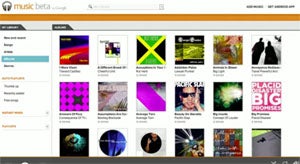This image is a screenshot of Google's Music Beta website. The screenshot appears slightly blurry and pixelated, suggesting it is quite dated. The Music Beta service was one of Google's first forays into the music subscription market, likely aimed at early adopters and initial users. The website's layout is indicative of an older design, possibly from the early 2000s, which adds to its dated appearance.

The main page features 18 album covers across various categories, although the blurriness makes the specific categories and album titles indiscernible. None of the albums are recognizable, reinforcing the notion that this is an older version of the site. The design of the webpage includes elements that are less sophisticated compared to modern music subscription services, indicating that it was an early attempt to cater to music enthusiasts by allowing them to create playlists and explore music.

Overall, the screenshot provides a nostalgic glimpse into Google's initial attempts at establishing a music streaming and subscription service through their Music Beta platform.